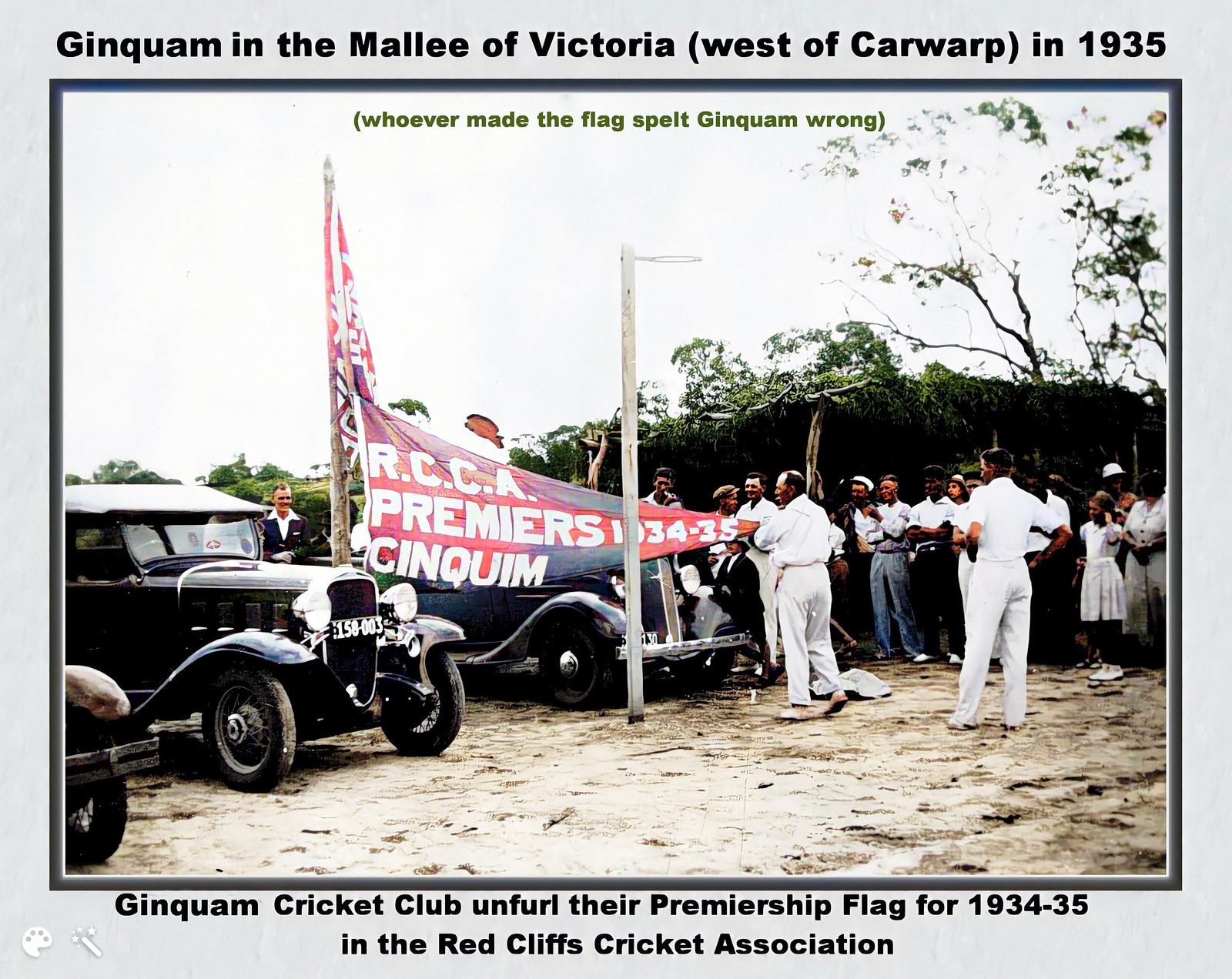This black-and-white photograph portrays the historic moment when the Gingquam Cricket Club proudly unveils their premiership flag for the 1934-35 season, under the auspices of the Red Cliffs Cricket Association. The image captures a nostalgic scene featuring vintage 1930s vehicles on the left, contributing to the authentic period atmosphere. Central to the image is a prominently displayed banner that reads "RCCA Premier 1934-35 Gingquam" in elegant white lettering against a backdrop of red and blue. This banner is being unfurled by a gentleman, dressed impeccably in white, standing in a large field that appears sparse in grass. The background showcases a picturesque hill adorned with trees and greenery, adding a vivid contrast to the otherwise barren field. A small but attentive crowd gathers to witness the event, highlighting the communal pride and significance of this achievement in the local cricketing history.